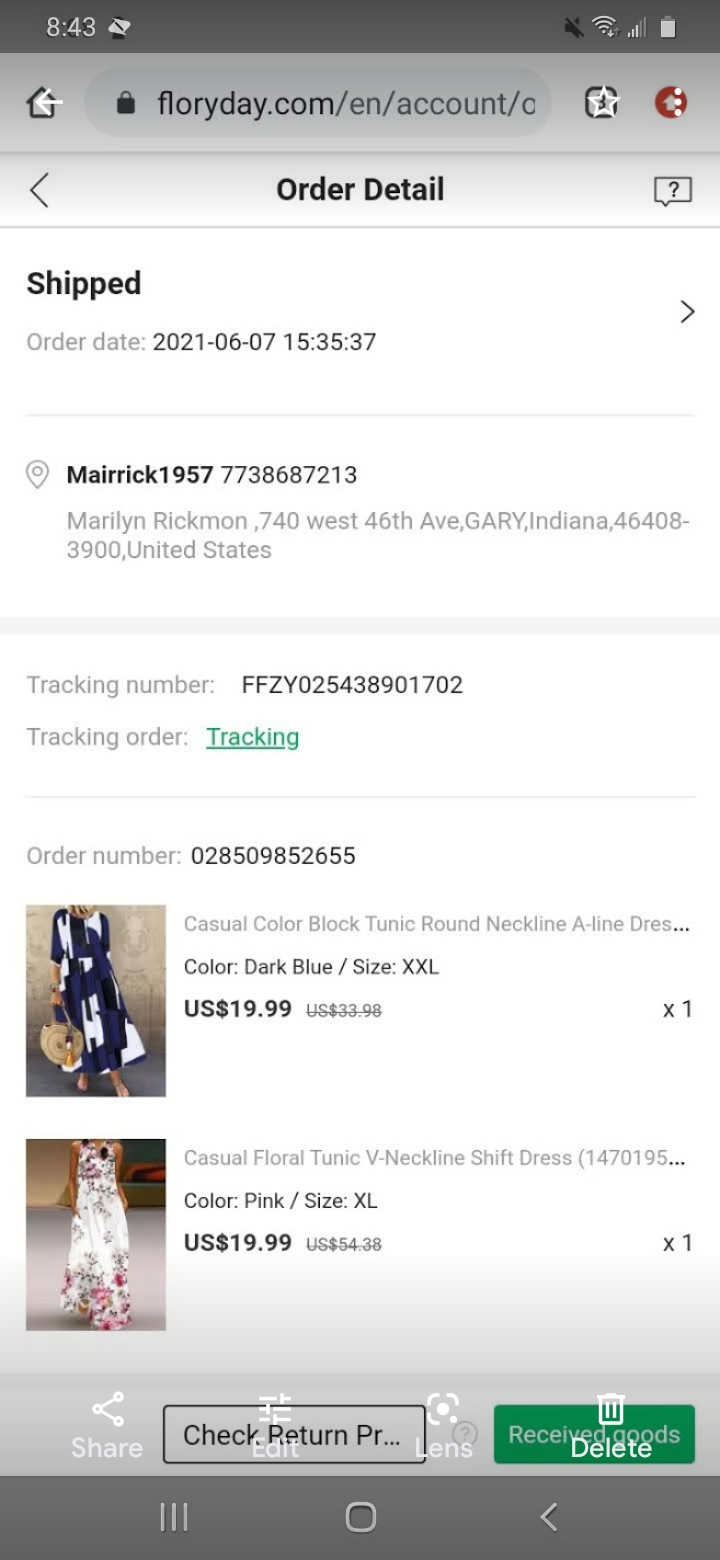A screenshot is depicted from a smartphone capturing various details typically seen on a mobile device's screen. The header displays a gray border showcasing the time as 8:43, alongside a distinctive emblem representing a white diamond inside of a black box. Toward the top right, familiar icons are present including a black icon denoting the phone signal strength, a battery icon indicating it is three-quarters full, and other standard symbols.

Beneath the header is a grayed-out horizontal bar featuring a black-bordered house icon accompanied by a white arrow pointing left. Adjacent to this is an oval search bar containing a black lock icon and the URL "floriday.com/en/account/c" in black and gray text, followed by a black box with a white star, a red circle with a gray dot, and three white dots to the right.

The layout continues with a black arrow pointing downward and a lighter gray section inscribed with "Order Detail" in black, beside a gray box with a question mark. A thin horizontal gray line divides sections, followed by the word "Ship" in black text with additional order details such as "Order Date: 2021-06-07 15:35:37" next to a right-pointing black arrow. Another gray line demarcates further information below.

Listed next is contact information featuring "Merrick 1957" in black, accompanied by a phone number "773-868-7213". Below this, "Marilyn Rickman" is mentioned with an address "740 West 46th Av, Gary, IN 46408-3900, United States".

Further details include "Tracking Number: FFZY-025438901702" in black text, with "Tracking Order" in green beneath. The order number "028-509-852655" is displayed, followed by a rectangular picture of a woman in a black dress with white patches, holding a tan purse. The description beside reads "Casual Block Tunic Round Neckline Dress" with specifications including "Color: Dark Blue" and "Size: XXL". The price is marked as $19.99 with a previous price $33.98 crossed out, quantity indicated as "x1".

Another image shows a woman in a white dress with reddish floral patterns, described as "Casual Floral Tunic V-Neckline Shift Dress (1470195)", with details specifying "Color: Pink" and "Size: XL". The price is listed as $19.99 with a previous price $54.38 crossed out, quantity marked as "x1".

At the screen's bottom, a grayed-out rectangle contains icons such as a "Share" button with circles at its tips, an "Edit" function, and "Check Return PR" abbreviated, plus an icon resembling a lens labeled "Lens". Another icon shows a trash can symbol labeled "Delete". The very bottom has a gray bar with three white lines, a rounded square, and a right arrow pointing left.